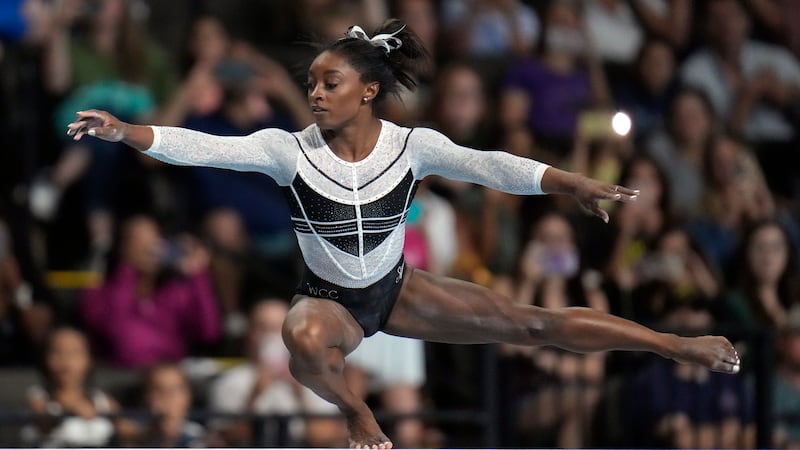This photograph features the renowned African-American gymnast, Simone Biles, captured mid-performance. She is showcasing an intricate acrobatic move, balancing on one bent leg with the other leg and both arms elegantly outstretched. Simone is attired in a striking black and white leotard, complemented by a white bow securing her hair. Her nails, both fingernails and toenails, are painted white. The blurred background reveals a crowded arena with an audience intently watching and taking photos, some visible with phone flashes. Though the beam she's performing on isn't visible due to the cropping of the image, the intensity and precision of her stance suggest she's engaging in a high-level gymnastics routine. The focus remains sharply on Simone, capturing her grace, strength, and focus in this extraordinary moment.